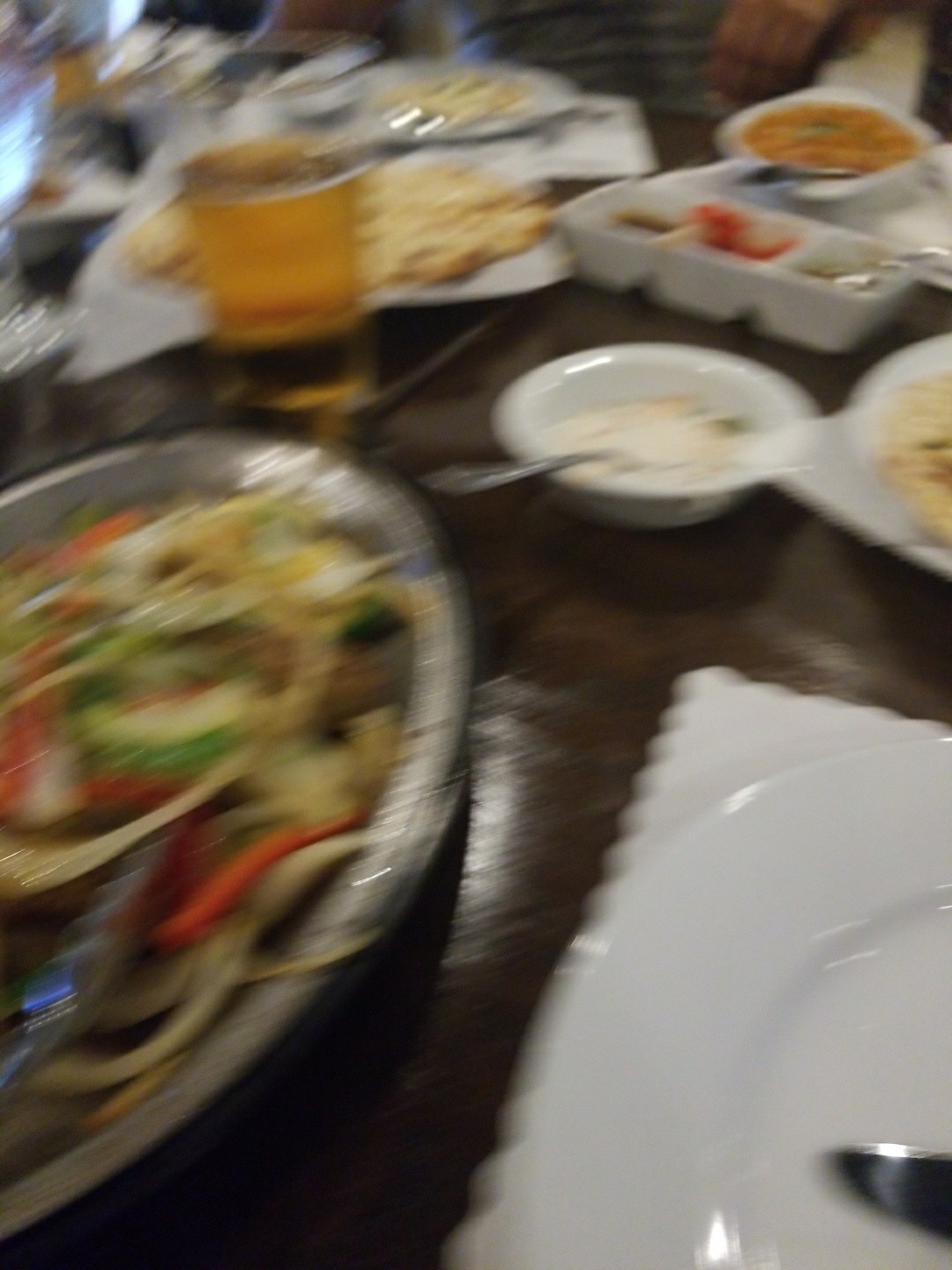In this somewhat blurry photograph, taken at what appears to be a bustling restaurant, a brown wooden table is filled to capacity with a diverse array of food and drink. Dominating the scene are multiple round bowls, plates, and various dishes, suggesting a group dining experience. Located toward the left-hand side, a silver round pan contains what looks to be stir-fried vegetables or fajitas, featuring vibrant colors of red, green, and brown. Adjacent to this dish, a frothy glass of beer stands prominently. Scattered across the table are smaller bowls and plates containing an assortment of appetizers, sauces, and toppings, with one notable white bowl filled with a white liquid and spoon. Despite the blur, the colorful spread of food items and the unending variety indicate a lively meal in progress, capturing the essence of communal dining.